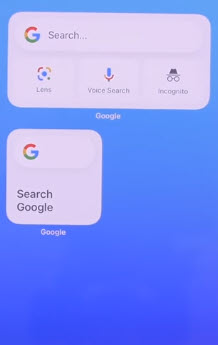The image depicts a heavily stylized dark blue background with white text and various branding elements reminiscent of a Google search interface. The top margin, as well as the left and right margins, are each about half an inch, framing the content centrally.

Approximately one inch from the top, left, and right edges lies a prominent gray rectangle occupying nearly the entire width of the image and extending vertically for about two inches. 

At the very top of this rectangle, a search bar stretches horizontally. On the left of this bar is the distinctive Google "G" logo, segmented with colors: yellow on the upper left, red on the lower left, green on the upper right, and blue on the lower right. Adjacent to this logo is the text "Search..." in black, indicating a placeholder for search queries.

Beneath the search bar, there are three aligned icons. The first icon is the Google Lens symbol, labeled "Lens" in black text below it. Next is the microphone icon representing Google's voice search, followed by the label "Voice Search." The third icon signifies incognito mode, accompanied by the label "Incognito."

Further below in the blue section of the image, the word "Google" is prominently displayed at the center in white text. Just to the left, there is a smaller square graphic featuring the Google "G" in the top-left corner. Below this "G" within the same square, the word "search" appears in black, followed by "Google." Outside this square and aligning with the second "G" in "Google," the word "Google" appears again in small white letters.

From this point downward to the approximately three-inch boundary at the bottom of the image, the background remains uniformly blue, completing the design.